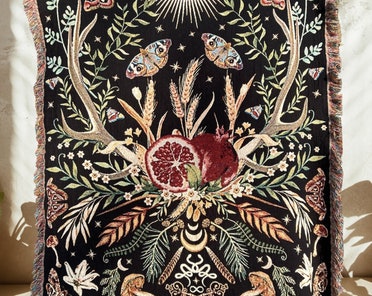A detailed image description combining all three captions:

The image depicts a richly textured rug hanging against a black background, serving as an eye-catching centerpiece with a striking symmetrical design. In the exact middle of the rug, contrasting its dark backdrop, is a deep red-colored pomegranate, presented both halved and whole. The half-cut pomegranate reveals its intricate interior, while the intact fruit beside it shows a noticeable stem. Emanating from this central motif are tan-colored branches and large elk antlers, giving it an elaborate, naturalistic framework.

Surrounding the pomegranate are various off-white and golden flowers, some with subtle orange or yellow centers, adding delicate detail to the vibrant composition. The top center of the image features a pair of moths, flying above the antlers, while two additional butterflies can be seen higher up, enhancing the sense of symmetry. At the very top, rays that resemble sunlight beams down onto the arrangement, adding a touch of luminosity.

Around the border of the rug, there are gold frills and frays, enhancing its ornate appearance. The surrounding artwork also includes elements like mushrooms, additional flowers, and leaves, contributing to the lush, nature-inspired tapestry that blends elements of flora and fauna seamlessly.